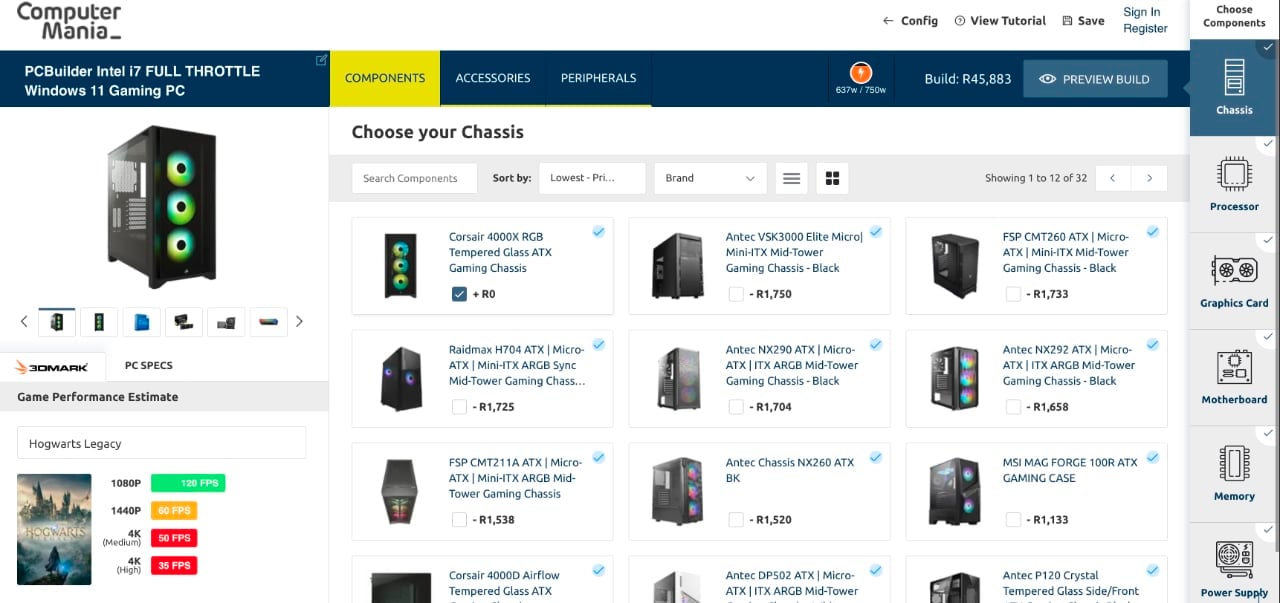The image features a detailed layout of an online PC builder interface. On the left-hand side, the top section in black is labeled "Computer" with "Mania" followed by an underscore underneath. On the right-hand side, there's a black arrow pointing left, labeled "Config." Below this arrow, the labels "Review Tutorial," "Save," "Sign In," and "Register" are displayed, with "Sign In" and "Register" highlighted with a black background.

The background transitions to teal, with "PC Builder" written in white on the left side and "Intel i7 Full Throttle" beneath it. Below these titles, it says "Windows 11 Gaming PC." A small yellow background highlights the word "Components" in black text. The background shifts back to teal with the words "Accessories" and "Peripherals" underlined in white.

Further down, there's a mostly orange circle with a white lightning bolt inside and a white outline. Below this, there's text in white: "637W / 750W." Another set of text reads "Build... R45,883," followed by a teal box labeled "Intel" and "Preview Build."

A pop-up pointing towards "Preview Build" is labeled "Choose Components." This overlay lists "Chassis" in white against a light gray background, then continues with "Processor," "Graphics Card," "Motherboard," "Memory," and "Power Supply" in the same color. Accompanying each label are images of the items, shown with various prices denoted by "R," though the specific currency is unspecified.